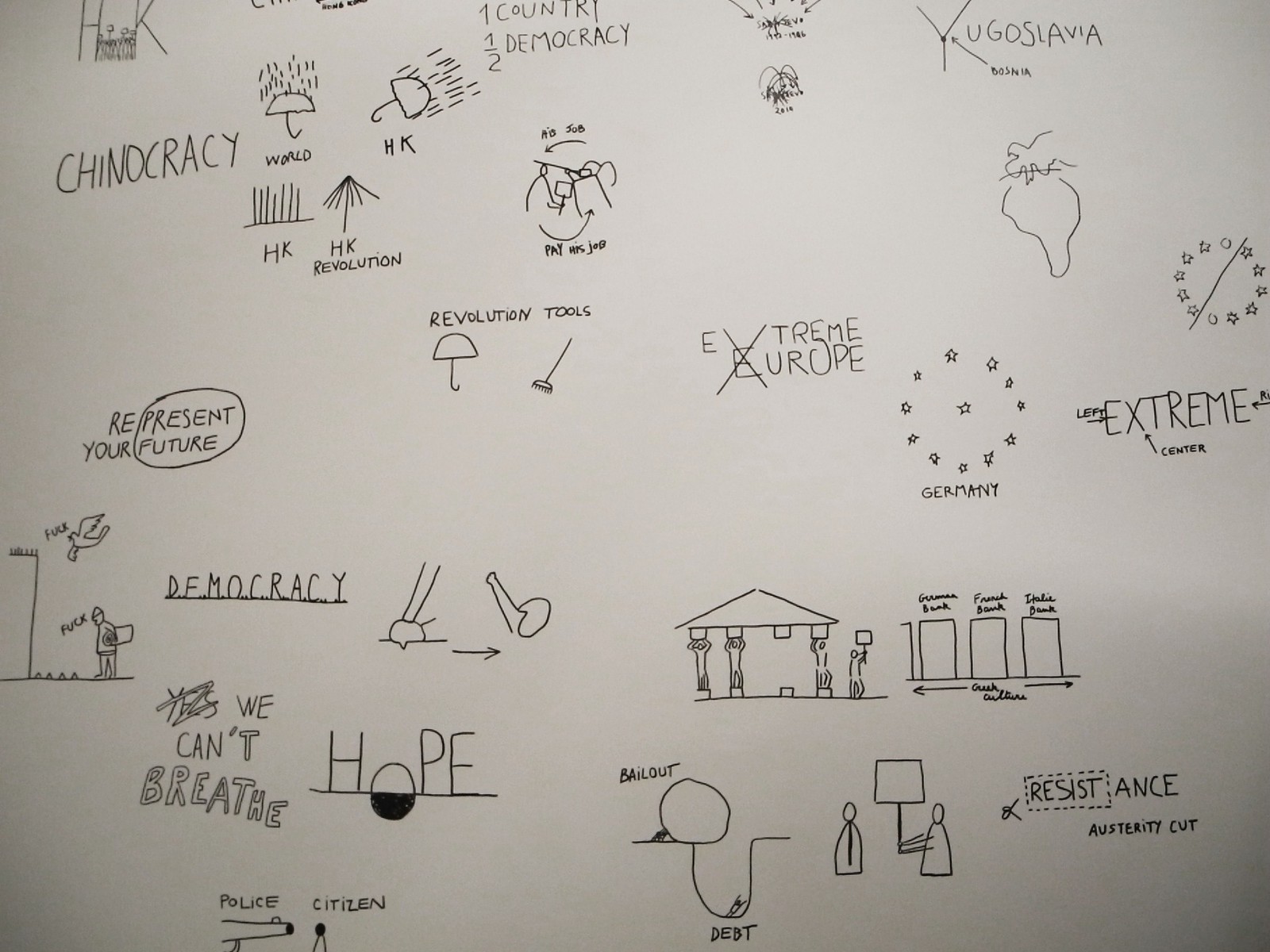The image features a grayish-beige background filled with a variety of hand-drawn illustrations and text that express political sentiments and social commentary. Prominently, several umbrellas are depicted: one to the left with the word "world" under it and "China Chrissy" written nearby, while another to the right has "HK" at the bottom. The upper left corner showcases "HK" with grass beneath, along with "China Crossy" and an umbrella with rain. 

Key phrases are scattered throughout the image, such as "democracy," "we can't breathe," and "hope." There are also recurring themes of revolution, with words like "HK revolution" and imagery of protest tools like an umbrella and a rake labeled "revolution tools." The word "hope" is prominently drawn, symbolizing an optimistic outlook amidst the protest themes.

Notable imagery includes a bird and a walking man, both saying "F-U-C-K," and a scene depicting a citizen with a gun pointed at him by the police. The phrases "represent your future" and "present future" are circled, emphasizing the protest's focus on the impact of the current events on the future.

In addition, broad geopolitical references such as "Yugoslavia and Bosnia," "Europe extreme" with a crossed-out "E," and "Germany as a star" surrounded by other stars appear to map the context of global resistance movements. The mention of "country have democracy" further ties the local themes to a larger, global struggle for democracy.

Overall, the image is a detailed, politically charged collage of text and drawings reflecting the sentiment and tools of a protest for democracy and social justice.